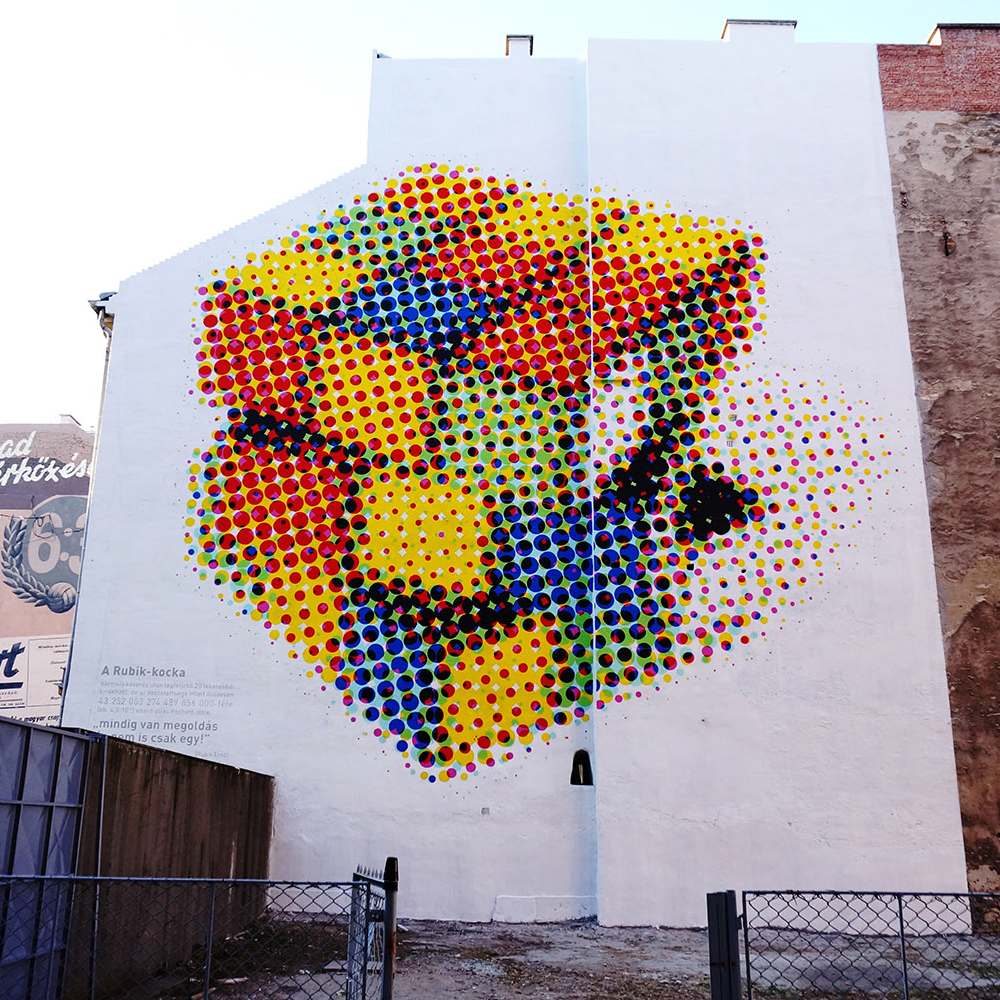The photograph captures an urban scene with a large mural adorning the side of an unconventionally shaped building. The mural's background is white, prominently featuring an abstract representation of a Rubik's Cube rendered in a dot matrix style. The Rubik's Cube appears slightly twisted, with its various levels angled differently. The colors in the cube span from red, orange, yellow, green, and blue to black, creating a vibrant, shadowed effect. Below the Rubik's Cube is text that reads "A RUBIK KAKA." The scene also includes a commercial trash dumpster beside the building and a black metal fence with an open gate in the foreground. In the distance, there is cursive writing on a building with an umlaut over an 'o', suggesting the location is likely Germany. The ground near the building is dirty and unkempt, and a brown wooden fence is visible on the left side of the image.